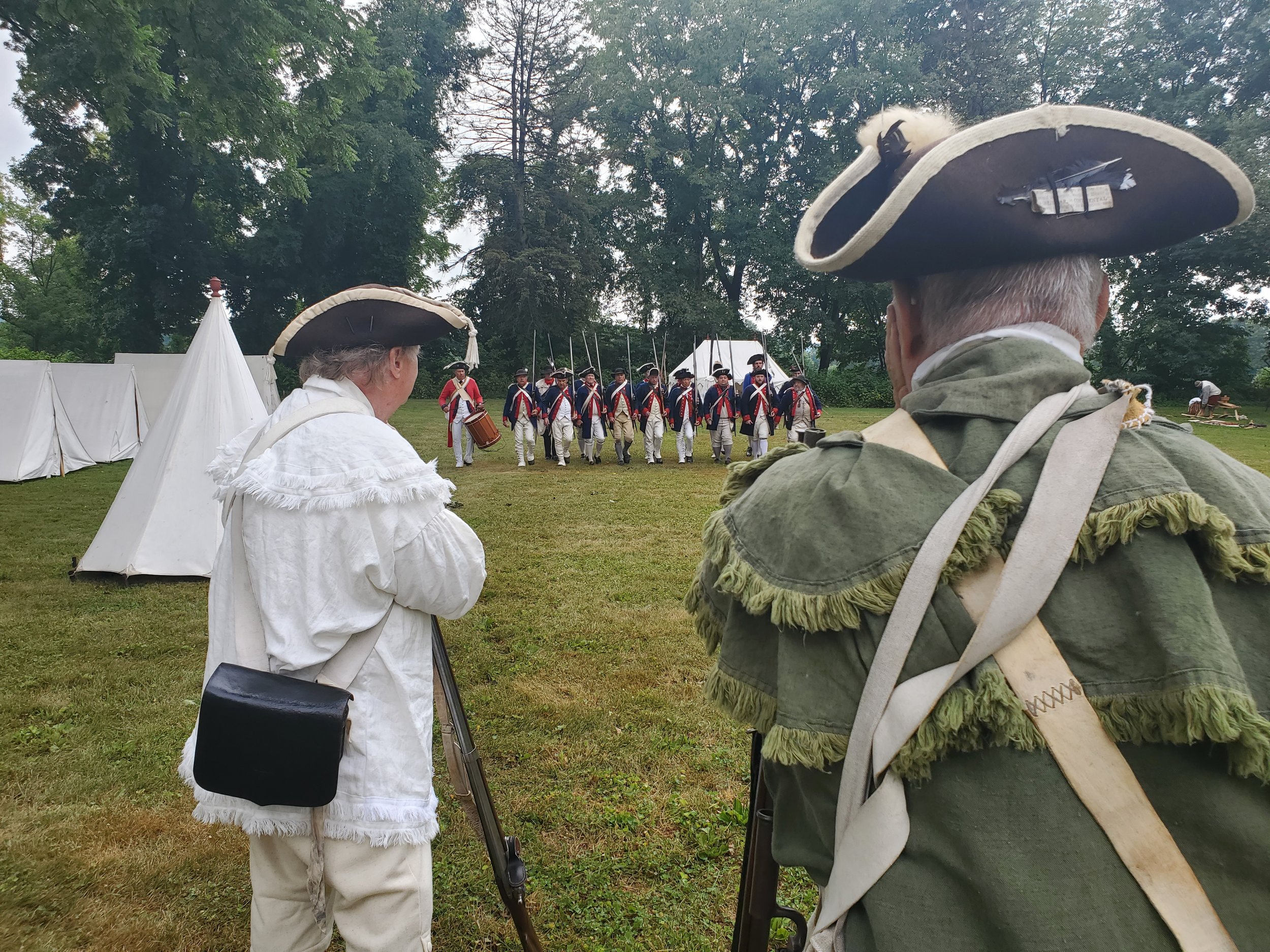In this detailed photograph of a Revolutionary War reenactment, a group of reenactors is assembled on a spacious grass field surrounded by green trees and a sky seen through the branches. On the right side of the image, a man dressed in an olive green coat with a double-layered fringe collar stands facing away from the camera. He has gray hair and a white canvas strap crossing from his left shoulder to his right, and another strap from his right shoulder to his left, supporting the rifle he holds upright in front of him. His black and white tricorn hat aligns with the era's style. To his left, a man in a white fringed jacket, beige pants, and a similar tricorn hat stands with a black bag slung across his body, also holding a rifle upright.

In the middle distance, a troop of men in dark blue jackets with red trim, white shirts, and pants march forward. They carry rifles upright and match each other in their black and white hats. One of these men, distinguished by his red jacket, pounds a drum, leading the troop. On the left side of the image, several white canvas tents, one resembling a teepee, are positioned, adding to the authentic period setting. In the background, more white tents are partly visible behind the marching troop, completing the historical tableau.